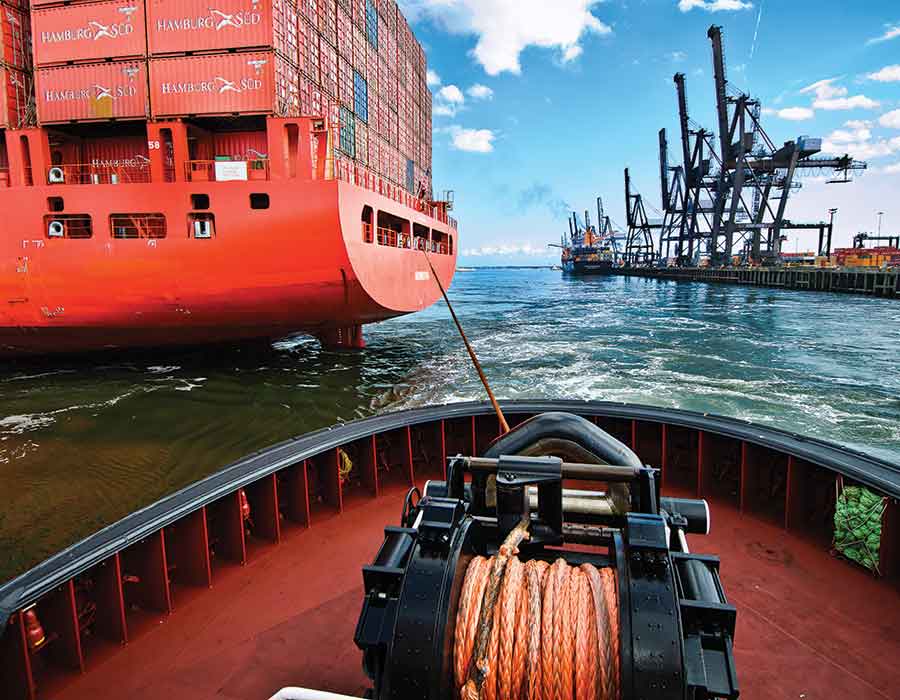A clear photo taken on a sunny day with a few fluffy clouds showcases an outdoor harbor scene. The perspective is from the deck of a red tugboat, which is being pulled by a much larger red cargo ship positioned to the left. An eye-catching thick orange rope, managed by a black winch on the tugboat, connects both vessels. The cargo ship stands tall, towering above the tugboat with six visible rows of red and sporadic blue cargo containers, stacked high and stretching about ten containers across. The water in the harbor is a darkish green, peacefully reflecting the blue skies above. The backdrop includes a bustling dock area filled with more shipping containers and large shipping cranes ready for loading, along with another cargo ship visible in the distance.